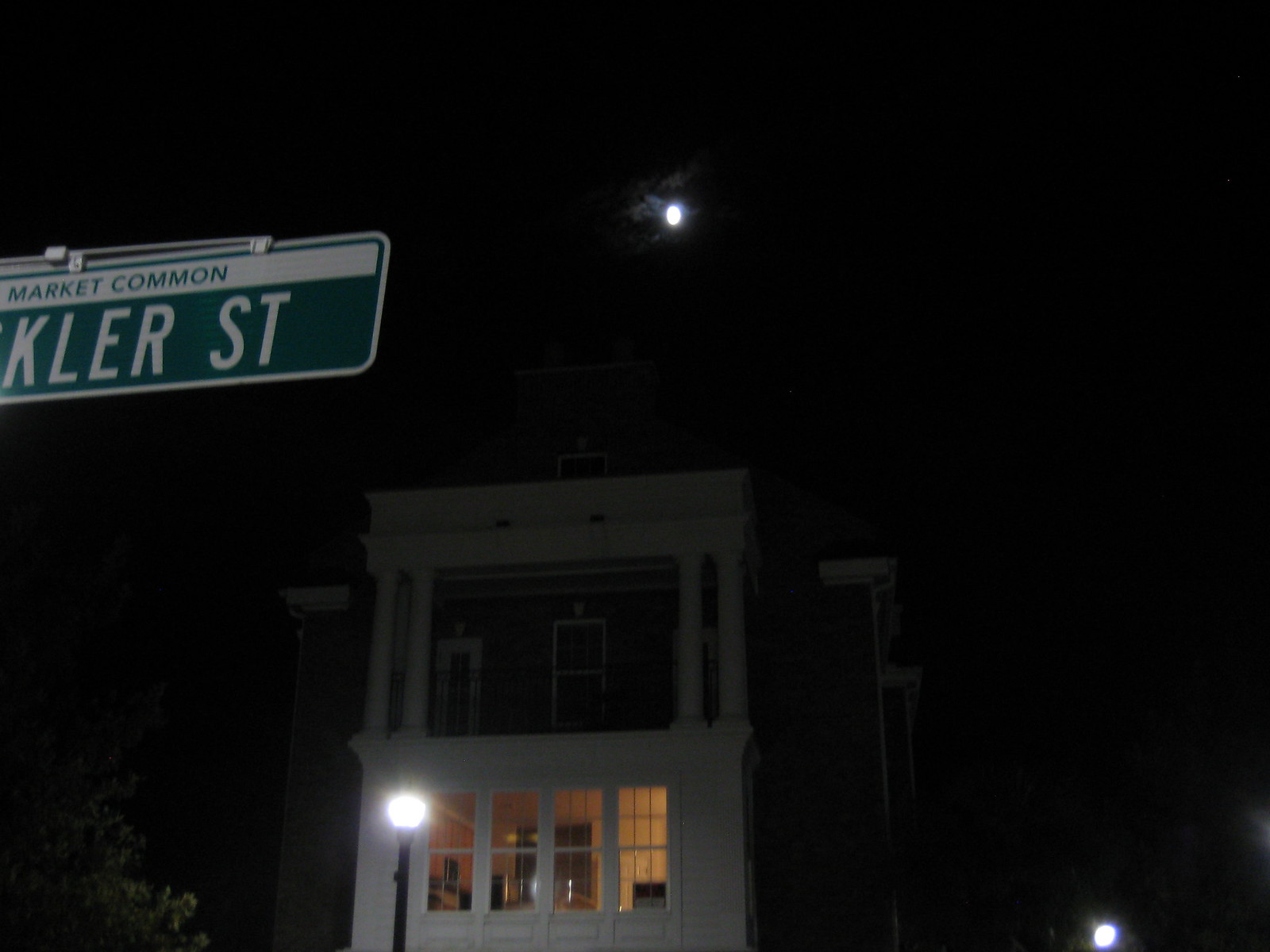The photograph captures a nocturnal street scene, focusing on a two-story house located near the street side. Prominently featured is a partially visible street sign that reads "Market Common," with an additional partial word "K-L-E-R" visible, although the first few letters are obscured. The house itself stands imposingly with its two stories; the upper floor includes a balcony, but details are obscured due to the lack of lighting. 

In contrast, the ground floor of the house is illuminated, hinting at a living room or similar interior space, though the interior remains indistinct. Above the house, a dark sky showcases a visible moon, casting a subtle glow. To the right, a street light provides additional illumination, blending with a house light that accentuates the entrance path. The entire scene is enveloped in the quiet stillness of night, framed by the darkness, with these few light sources punctuating the serene, shadowy ambiance.